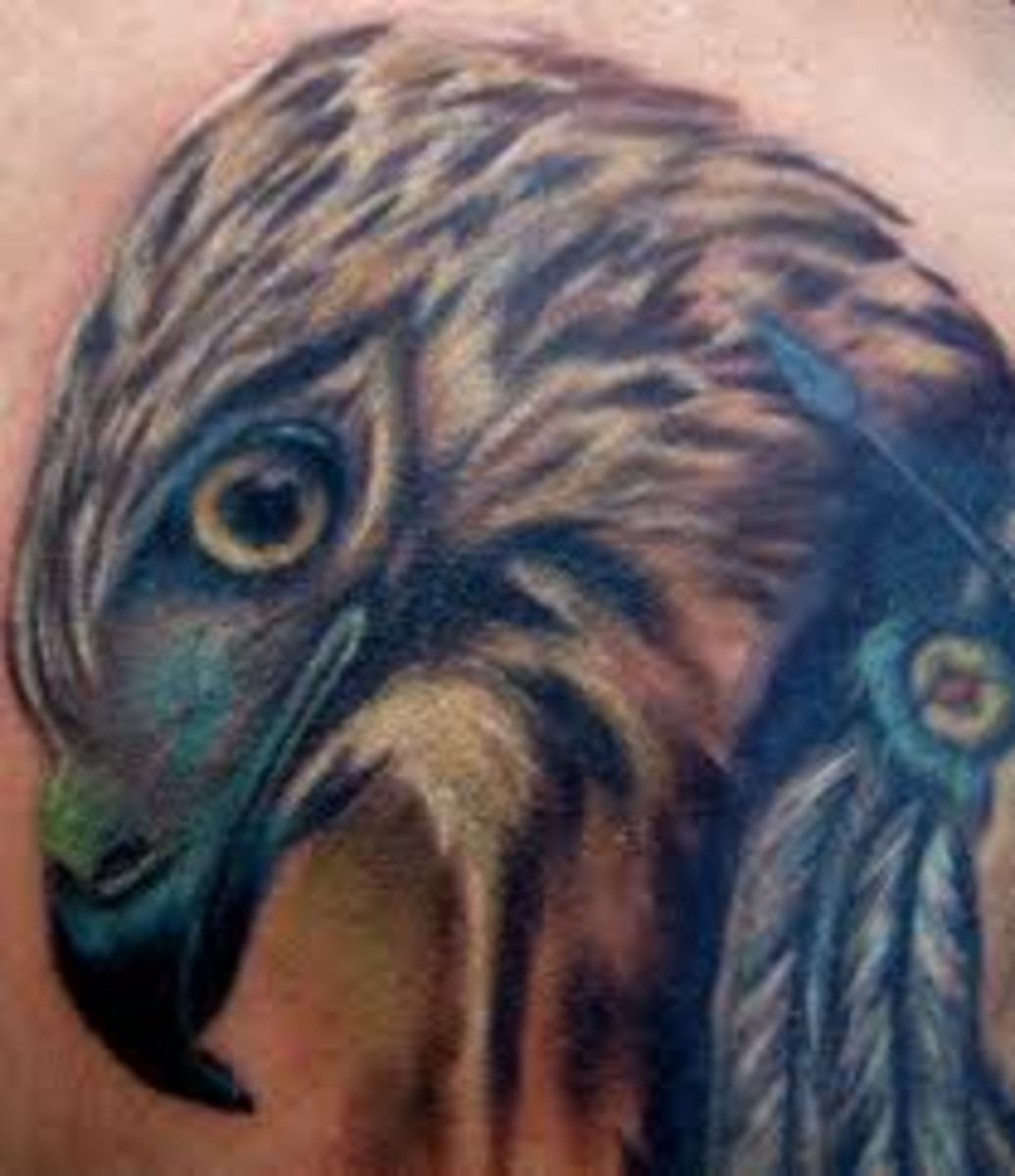The image depicts a detailed, close-up view of a tattoo on white skin, showcasing the head of a bird, possibly an eagle or hawk, in profile. The bird is facing to the left, featuring a prominently bronze eye, a beak that is green at the base and black at the tip, and an intricate mix of brown, gray, and black feathers. The tattoo includes additional artistic elements like Indian feathers and an arrow on the bird's neck, with a small yellow and blue emblem. The background appears flat, potentially in hues of pink or gray, giving the tattoo an undersaturated or filtered appearance. The focus remains on the bird's head with only a hint of the shoulder visible, emphasizing the intricate design and colors of the tattoo.